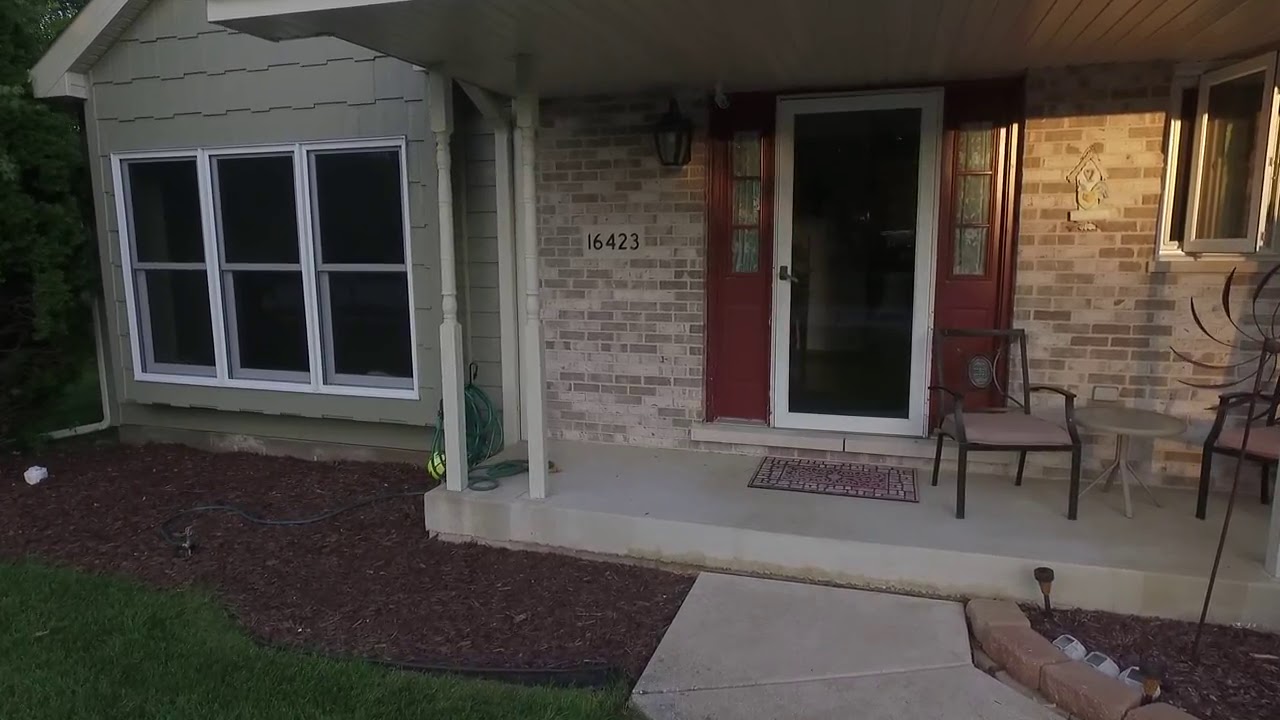In this image, we see the front exterior of a house with the house number 16423 displayed to the left of the door. The house features a combination of red bricks in varying shades from light gray to tan and light brown. The front yard includes a small patch of grass on the lower right and a landscaped area lined with bricks filled with mulch, primarily situated on the right side of the image.

The front door is a notable rust-colored wood, flanked by white aluminum trim, and it may have a screen door. On each side of the door, there are three sections of window panels, adding to the door's detailed appearance. To the left of the door, there's an additional white-paneled door with what appears to be a decoration shaped like a birdhouse mounted on the brick wall.

There are two chairs and a table on the small concrete patio at the front entrance, contributing to a cozy sitting area. You can also see a portion of the sidewalk leading up to the front patio and door. 

The upper left corner of the facade features three-sectioned windows, while the upper right includes a partially open window. There's a distinct addition on the left side of the house with a typical vinyl siding rather than brick. The main colors present in the scene are whites, greens, and various shades of tan and brown. No animals or people are visible.